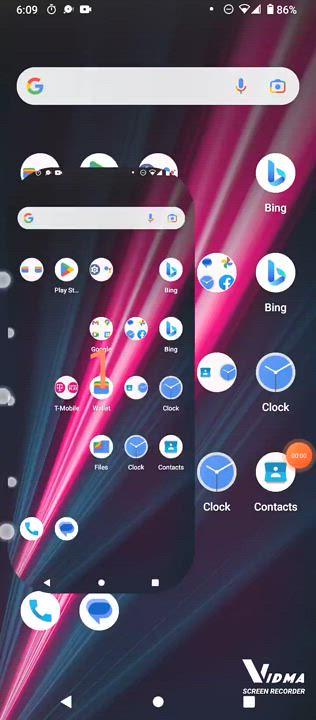The image is a screenshot of a smartphone, showcasing its home screen with distinct elements. Dominating the top section is a Google search bar, characterized by an oval shape. Within the search bar, the Google logo is located on the left, while icons for the microphone and Google Lens are on the right. The background is vibrant, featuring dynamic streaks or rays that emanate from the lower left corner, blending various shades of gray and converging into a cluster of pink and white in the center.

The home screen is arranged with a series of circular app icons. The left column includes two Bing icons, followed by a clock and a contacts icon. A successive row also features a clock icon. At the bottom right corner, the text "Vidma screen recorder" appears in white against a solid black background. Additionally, there is a smaller, inset image of the same home screen on the left side of the screenshot, indicating that a screenshot is being captured within the larger screenshot. The inset image is a precise duplicate of the primary screen layout. An orange notification bubble with the number "1" is visible, positioned next to the T-Mobile icon in the status bar.